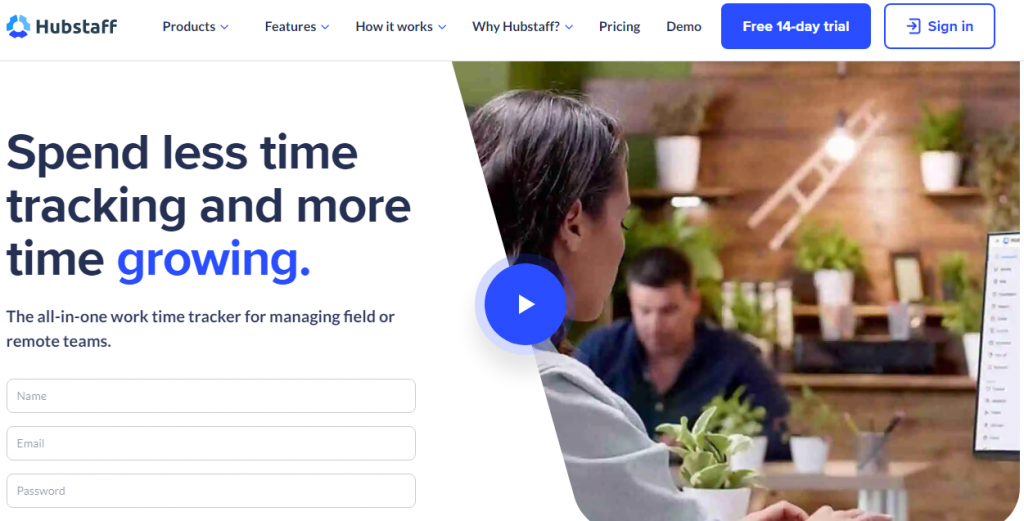The webpage features a clean and organized layout with a prominent white header at the top. Positioned in the top left corner is the Hubstaff logo, which comprises three different shades of blue in a circular design. To the right of the logo, "Hubstaff" is displayed in bold black text. Following this, several menu options are listed in non-bold black letters: 

- "Products" with a drop-down menu
- "Features" with a drop-down menu
- "How It Works" with a drop-down menu
- "Why Hubstaff" with a drop-down menu
- "Pricing" without a drop-down menu
- "Demo" without a drop-down menu

To the far right, there is a dark blue button labeled "Free 14 Day Trial" followed by a white "Sign In" button.

Beneath this header, on the left side of the page, the content is set against a plain white background with black text. The main headline reads "Spend less time tracking and more time growing," with the word "growing" highlighted in blue text. Below this, in smaller font, a subheading states, "There's only one work time tracker for managing field or remote teams." Following the subheading are three text boxes for user input: "Name," "Email," and "Password," intended for visitors to sign up or log in.